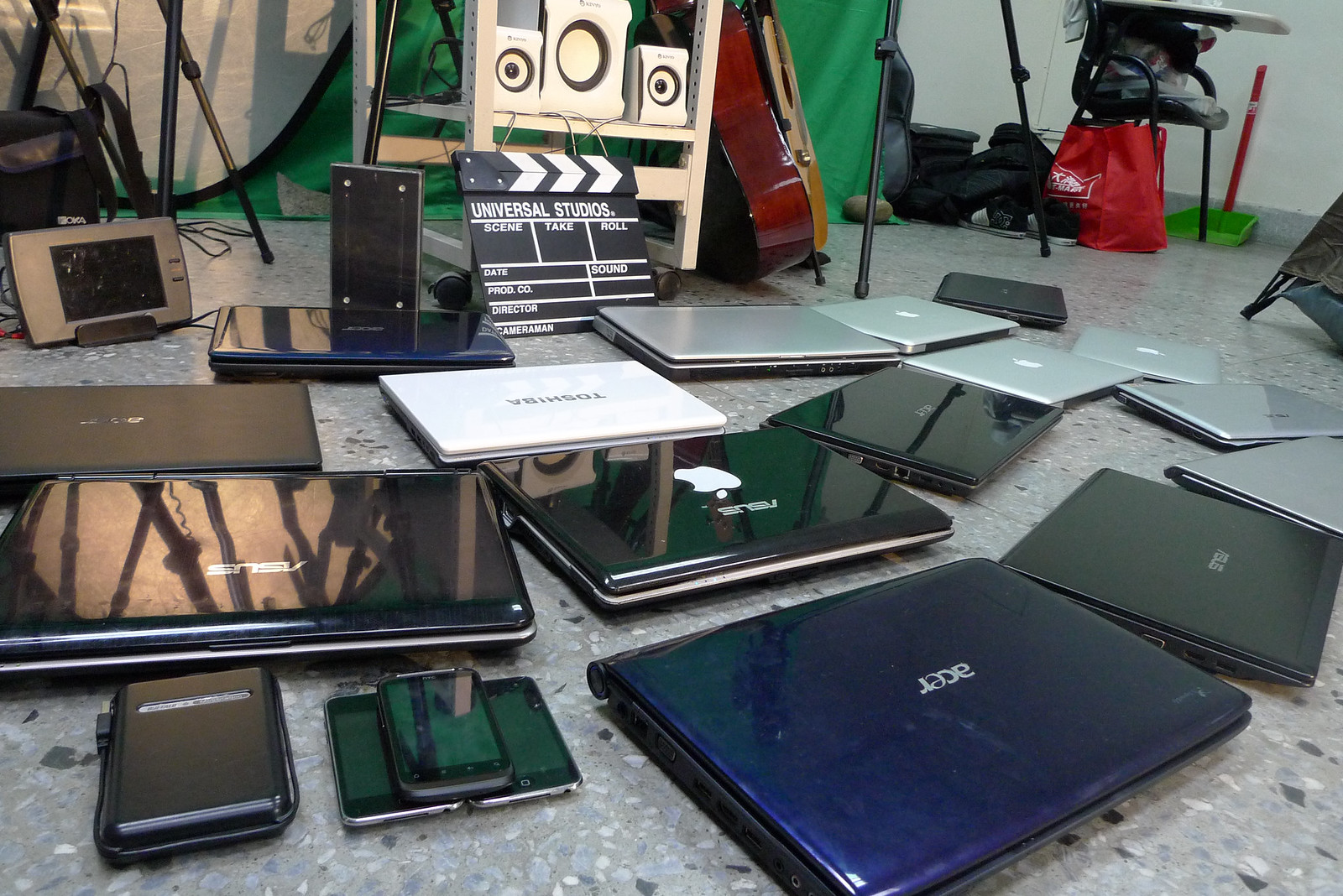This image captures a collection of 15 laptops arranged in an arch on a gray speckled concrete floor, resembling a cafeteria setting. The laptops are of various brands including Acer, Asus, Toshiba, and Apple, with colors spanning black, silver, blue, and a notable black Apple laptop with a distinctive white Apple logo. In addition to the laptops, there are three older smartphone models and a portable charger positioned at the bottom left of the image. The background features a Universal Studios clapperboard propped up on a white cart, flanked by two guitars—one red and one light brown—leaning against the right side of the cart. Further in the background, there are speakers, a green screen, containers, and a chair loaded with bags. The scene appears cluttered, suggesting a setting reminiscent of a movie set or a garage filled with various electronic and musical equipment.